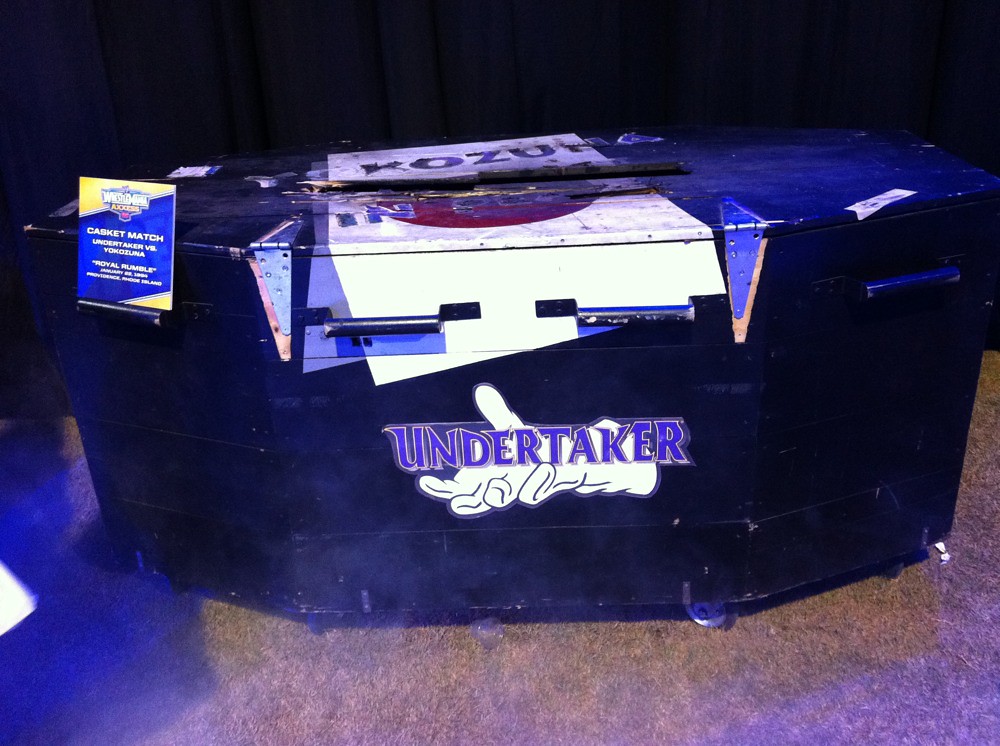In the image, we find a prominent wooden casket prominently positioned in the center, appearing to be part of the WWE arena setting. The casket, with its dark hues of black and wooden tones, features visible wear and splintering, suggesting it has been struck or impacted, particularly at its center. Across the bottom, the name "Undertaker" is emblazoned, attributing it to the famous wrestler. To the left of the casket, a poster reads "WrestleMania Casket Match Undertaker vs Yokozuna Royal Rumble." The background shows a dark curtain, giving an indoor, stage-like environment. The casket is equipped with handles, further emphasizing its coffin-like appearance, and adorned with details including the Undertaker's logo and possibly the remnants of a Japanese flag, reflecting its historical significance from a notable wrestling event. The color palette of the image is dominated by deep maroon, striking yellow, somber gray, and touches of blue and white, adding to the dramatic atmosphere of the depicted scene.